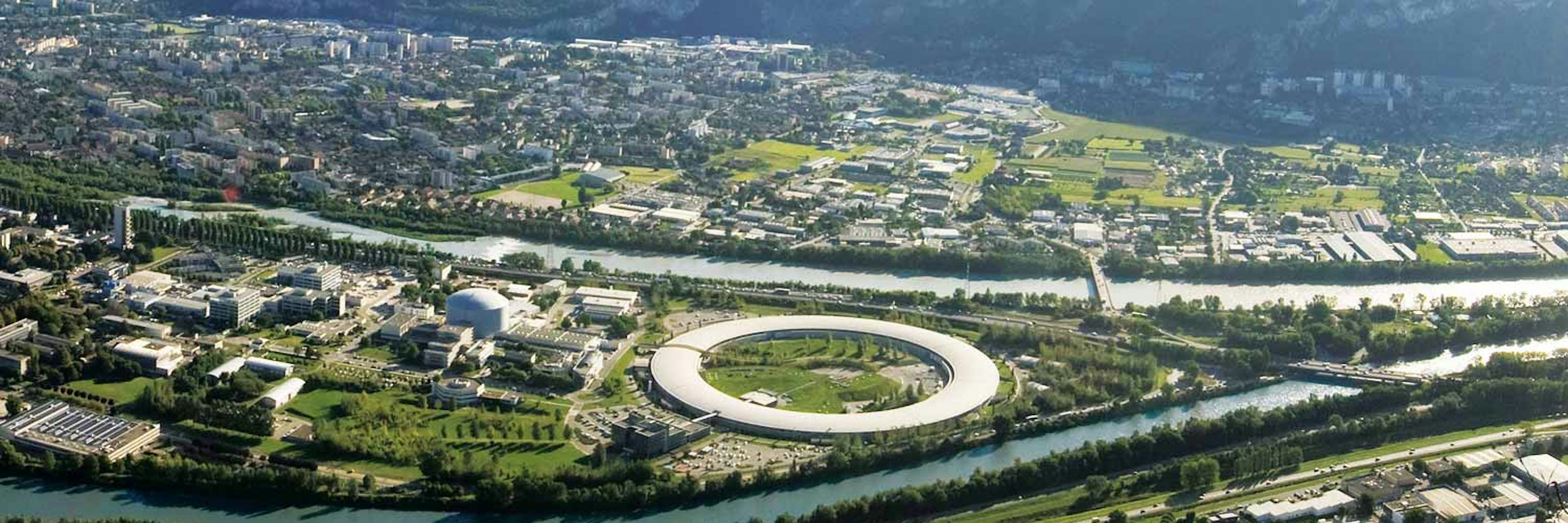This is a vibrant, panoramic aerial photograph of a sprawling city taken during the daytime. A noticeable haze, imparting a cyan tint, blurs some background details, adding a dreamlike quality to the scene. Dominating the center of the image is a distinctive, round, donut-shaped building situated beside a river that runs horizontally across the photograph. Above this structure, the river divides into two, flowing across the bustling cityscape. The city is a tapestry of greenery, white roofs, and gray structures, with dense clusters of buildings indicating a lively downtown area. A prominent highway cuts through, while the top right-hand corner reveals a shadow, perhaps cast by distant mountains. Patches of grass and trees intersperse the urban sprawl, enhancing the city's blend of natural and architectural elements.